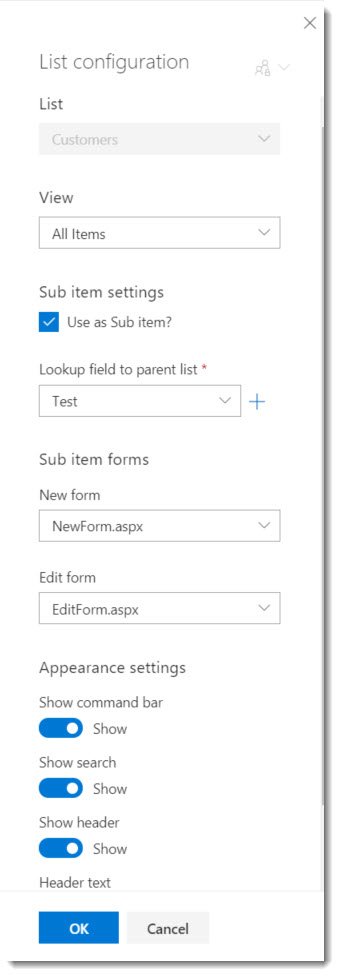This image is a detailed screenshot of a "List Configuration" panel, likely from a content management system or web application, designed for configuring lists. At the top of the panel is the header titled "List Configurations," clearly indicating the purpose of this section. 

The first element below the header is a dropdown list labeled "List," displaying the value "Customers." This dropdown is grayed out, suggesting it is not editable. Following this, there is another dropdown menu that seems to allow users to change the view of the list.

Below these dropdowns, there is a checkbox labeled "Use Sub-items," which is checked, indicating that sub-items are enabled for this list. Adjacent to this is a "Lookup Field to Parent List" dropdown, currently set to "Test." A small plus icon next to it indicates the option to add or configure lookup fields.

Further down, there are configurations for different forms associated with the list. The "Sub-item New Form" dropdown is set to "newform.aspx," while the "Edit Form" dropdown shows "editform.aspx," denoting the specific pages used for new item creation and editing existing items, respectively.

Also visible are toggles for various interface elements such as the command bar, search bar, header text, and action buttons. Each of these options is selected, indicating that they are active in the current configuration.

Overall, this panel allows users to configure various aspects of a list, including setting up different forms, adjusting views, and altering the appearance and settings of the list elements.